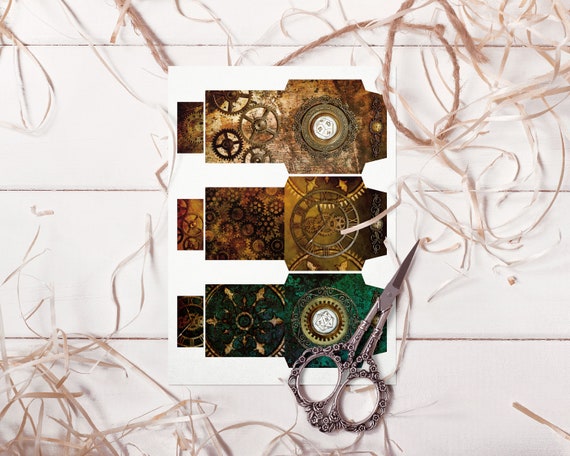In this intricate artwork set against a background of light gray to white wooden planks, thin strips of light brown and pink rope meander and scatter across the scene. Central to the composition is a vertical rectangular sheet of white paper, featuring three irregularly shaped, stacked images that resemble clockwork mechanisms, evoking the design of a traffic light. 

The topmost image prominently displays gold-colored gears and is positioned adjacent to a cluster of brown gears on the left. To the right of this, a gold-colored circle with a white center punctuates the arrangement. Below this formation, the middle image showcases a set of small, tightly grouped gears, with a visible clock mechanism on the right and an emerald-colored background underneath. A white circle surrounded by sun-like brown edges embellishes the center of this section.

Finally, the bottom image, bathed in a dark green hue, contains another circle framed by an emerald backdrop, which features clock numbers positioned around its perimeter. In front of this collection rests a pair of scissors with very small blades, remarkably large white finger holes, and decorative black and gray specks, adding a tangible, practical element to the otherwise mechanical setup. The entire arrangement rests upon a table constructed of white-painted wooden planks, enhancing the overall composition with a rustic charm.